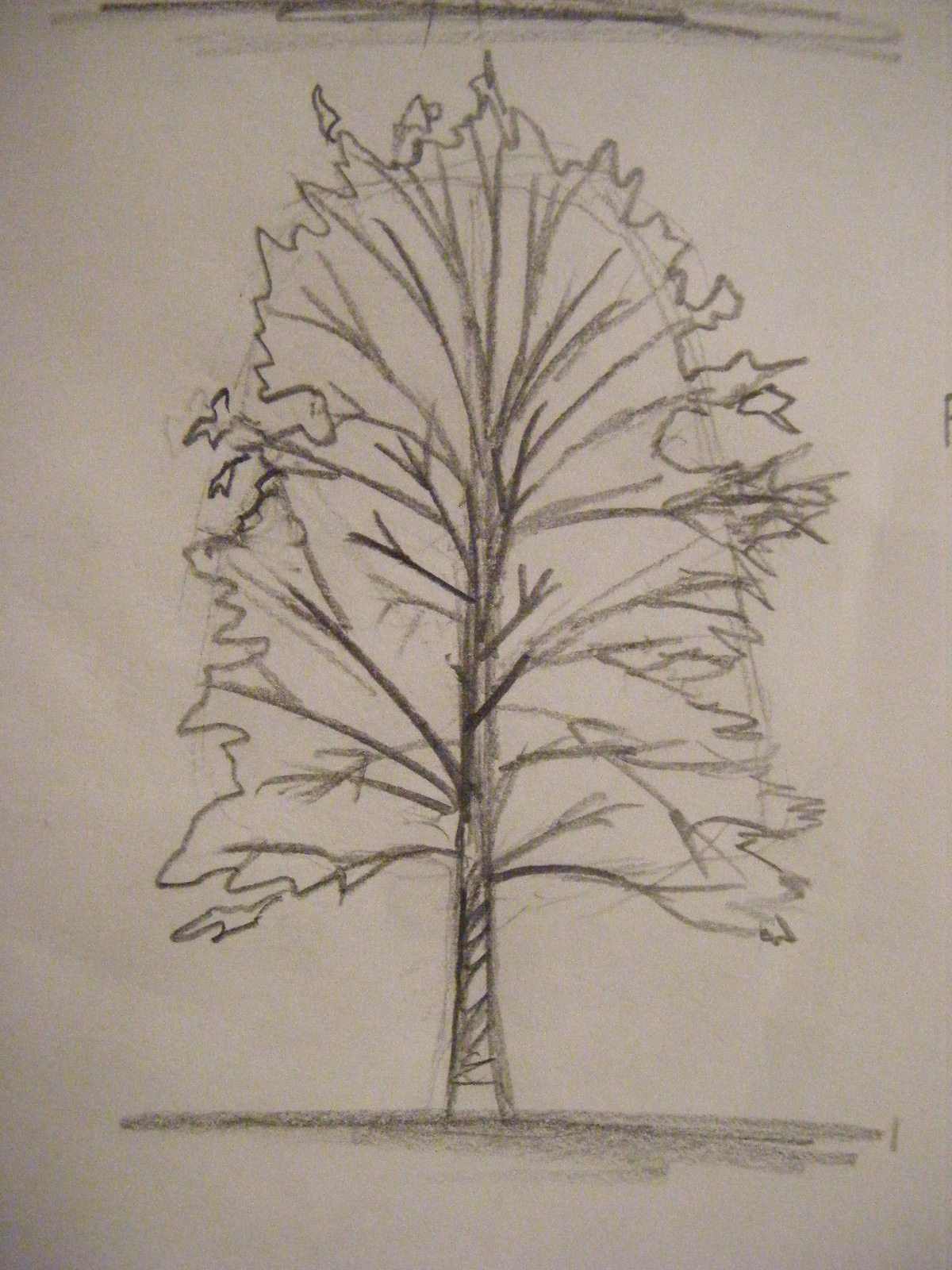This image portrays a detailed line drawing, resembling a child's artwork. The paper, under dim lighting, appears to have a greyish hue, though it might actually be white. Dominating the center of the composition is a tree with a tall, slender trunk, meticulously shaded with black pencil lines. Extending from the trunk, several branches stretch outwards, and the entire artwork is rendered in pencil. Encasing the tree, the drawing features a serrated border, imparting a somewhat rectangular frame to the image. Tiny elements, possibly depicted as leaves or even birds, delicately cling to the tree edges, appearing almost as if they might detach at any moment. At the base of the tree, horizontal pencil strokes suggest the ground, while a similar horizontal line at the top completes the scene. Noticeable creases run through the paper, particularly towards the middle right and left sections, adding texture to the artwork.